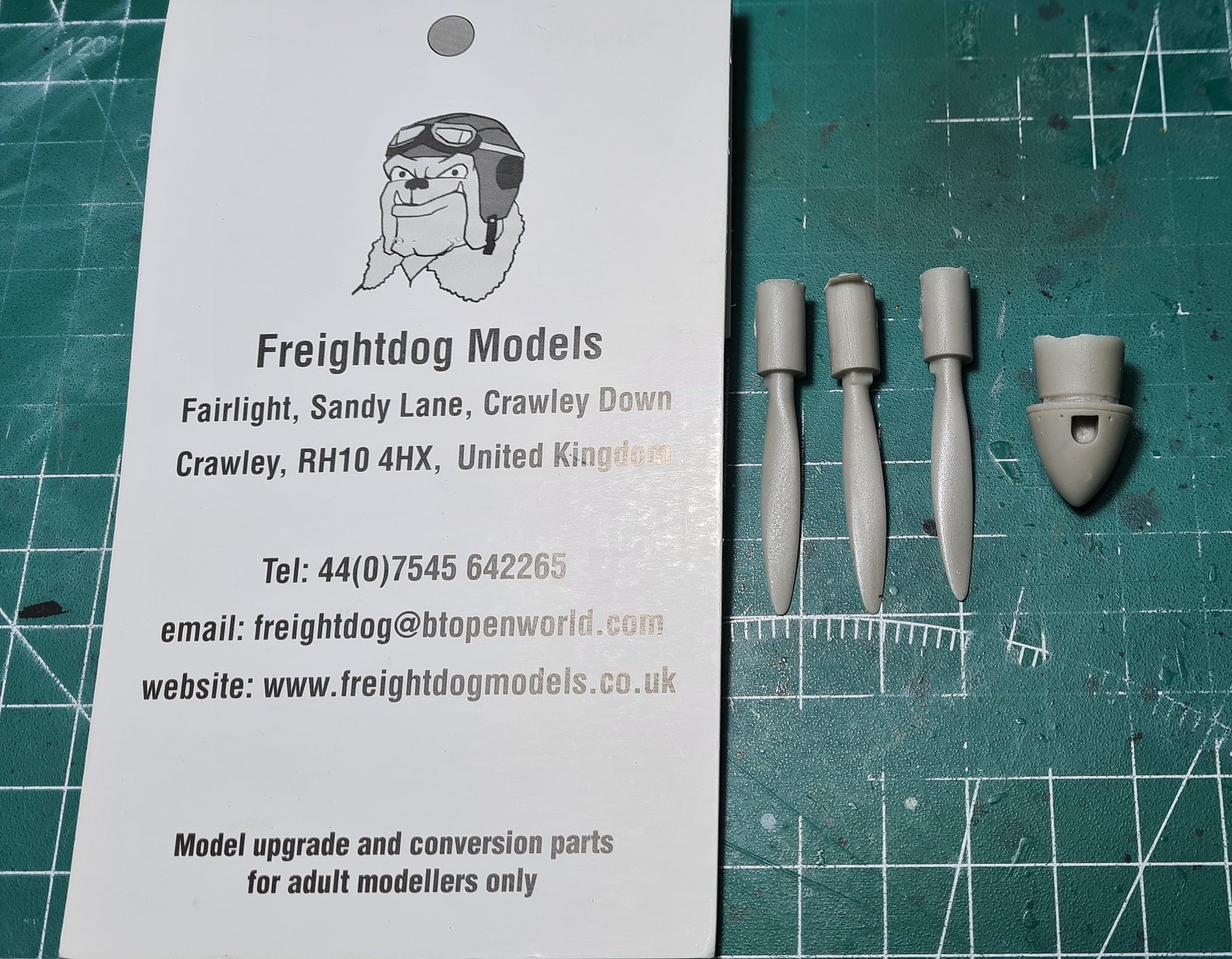The image captures a detailed display against a green backdrop designed like graph paper with white squares. On the left side stands a plaque featuring an illustration of an English Bulldog wearing an aviator hat and goggles, exuding a fierce expression with two fangs visible. The plaque reads: "Freight Dog Models, Fairlight, Sandy Lane, Crowley Down, Crowley RH10 4HX, United Kingdom." This is followed by contact information: "Telephone: 4407545642265, Email: freightdog@btopenworld.com, Website: www.freightdogmodels.co.uk." The bottom of the plaque states, "Model Upgrade and Conversion Parts for Adult Modelers Only." To the right of the sign, the display includes several gray plastic parts. Three of these parts are identical in size and shape, resembling propeller blades, while the fourth part has a distinct, bullet-like shape, clearly representing the tip where the propeller would attach on a model airplane.